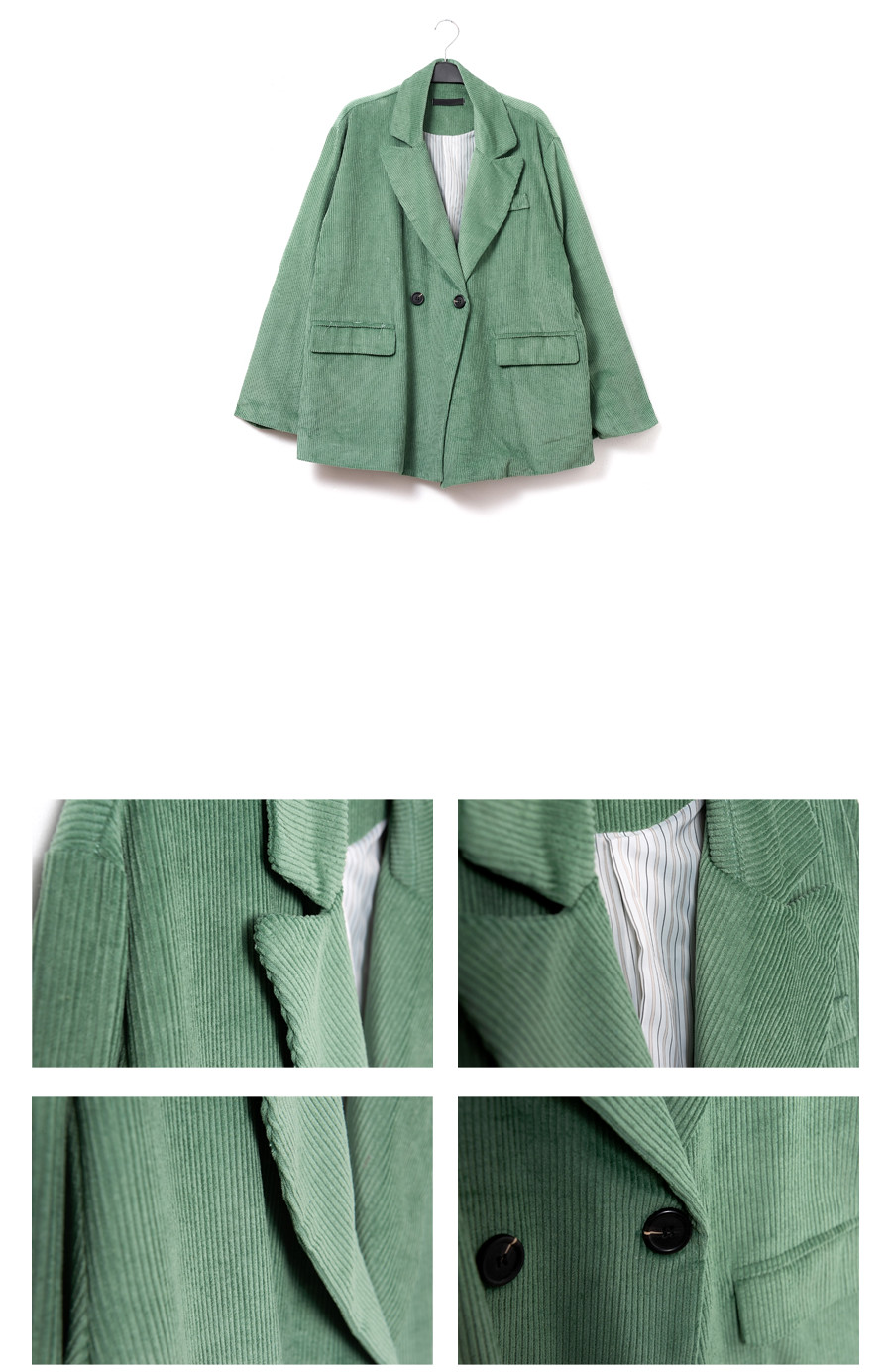The image is a detailed layout of a green corduroy blazer, depicted in a segmented format. The top part of the image showcases the entire blazer, with a color slightly darker than mint green, hanging on a clothes hanger as if for an online clothing ad. Below this are four separate close-up views arranged to form a larger rectangle. 

The blazer is double-breasted with two dark wood-tone buttons and features two lower front pockets. The inside is lined with white fabric featuring pinstriping. A white decorative shirt with stripes is visible underneath the blazer. The close-up images at the bottom provide detailed views of specific areas: the collar and sleeve, the collar and the underlying shirt, the bottom portion of the collar, and an up-close look at the two buttons. The blazer's texture is distinctly corduroy with a vertical pattern.